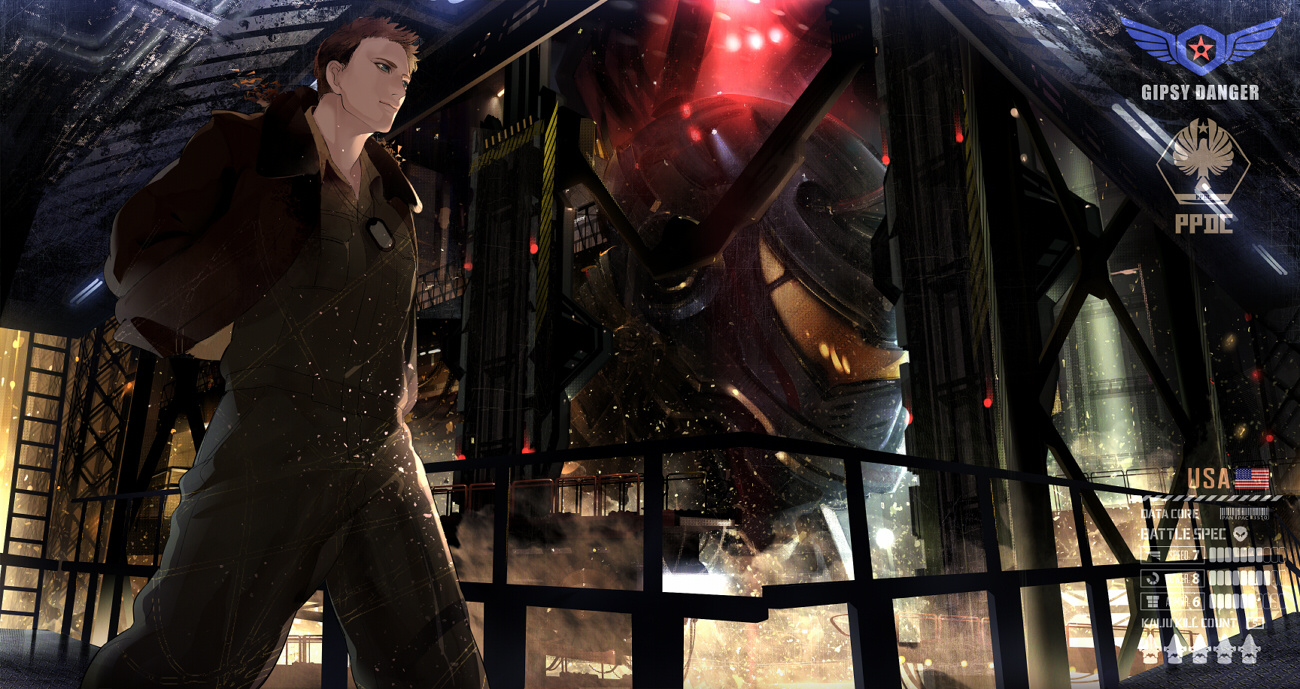The image appears to be a digitally-rendered scene from a video game or anime, featuring a strong, anime-styled male character with white skin and long hair, dressed in what looks like an olive or brown military suit. He stands prominently on the left side of the image. Behind him, there is a face of a giant mech, similar to those seen in anime, suggesting that he might be about to board or interact with it. The scene evokes a dark, gritty atmosphere, reminiscent of a dreary basement.

In the upper center of the image, there are noticeable red and pink lights, drawing attention immediately. To the upper right, there's a winged logo with an orange star, and beneath it, the text "Gypsy Danger". Further down, another symbol appears, featuring a hexagonal border and indistinguishable details. It is accompanied by the text "PPDC" and "USA" in orange, alongside an American flag and the outline of the USA map. The lower right corner displays various game elements such as bar levels representing different powers or items.

The background includes a slotted black fence or border with support posts, enhancing the military or industrial ambiance. The primary colors in the image are brown, yellow, black, blue, with accents of red, pink, and white, contributing to the overall dramatic and intense visual impact.